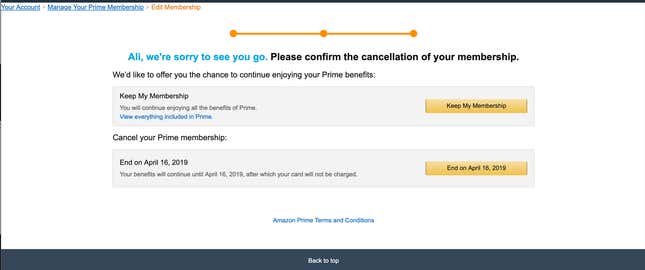This image is a screenshot of a webpage centered around the cancellation of an Amazon Prime membership. The rectangular screenshot has a white background with a black border. 

In the upper-left corner, there's a section labeled "Account" followed by four unreadable words in blue font and a word in orange font, where only "Edit" is legible. At the center of the top section, there is a line with three dots, positioned at each end and in the middle. Just beneath this, there's a blue text reading "We're sorry to see you go," followed by black text stating, "Please confirm the cancellation of your membership."

Below this message, there's a gray box with text that encourages users to retain their membership: "Keep my membership. You will continue enjoying the benefits of Prime," followed by more detailed benefits of Prime, though this text is partially obscured. Beneath this gray box, there's a prominent yellow button that says "Keep my membership."

Further down, there's another gray rectangle with the option to "Cancel your Prime membership on April 16th, 2019." Under this, there's text indicating that the benefits will continue until April 14th, 2019, with some additional unreadable words. Alongside this text, there's another button labeled "End on April 14th, 2019."

At the very bottom, "Amazon Prime" is mentioned again above a black bar that contains the text "Back to top."